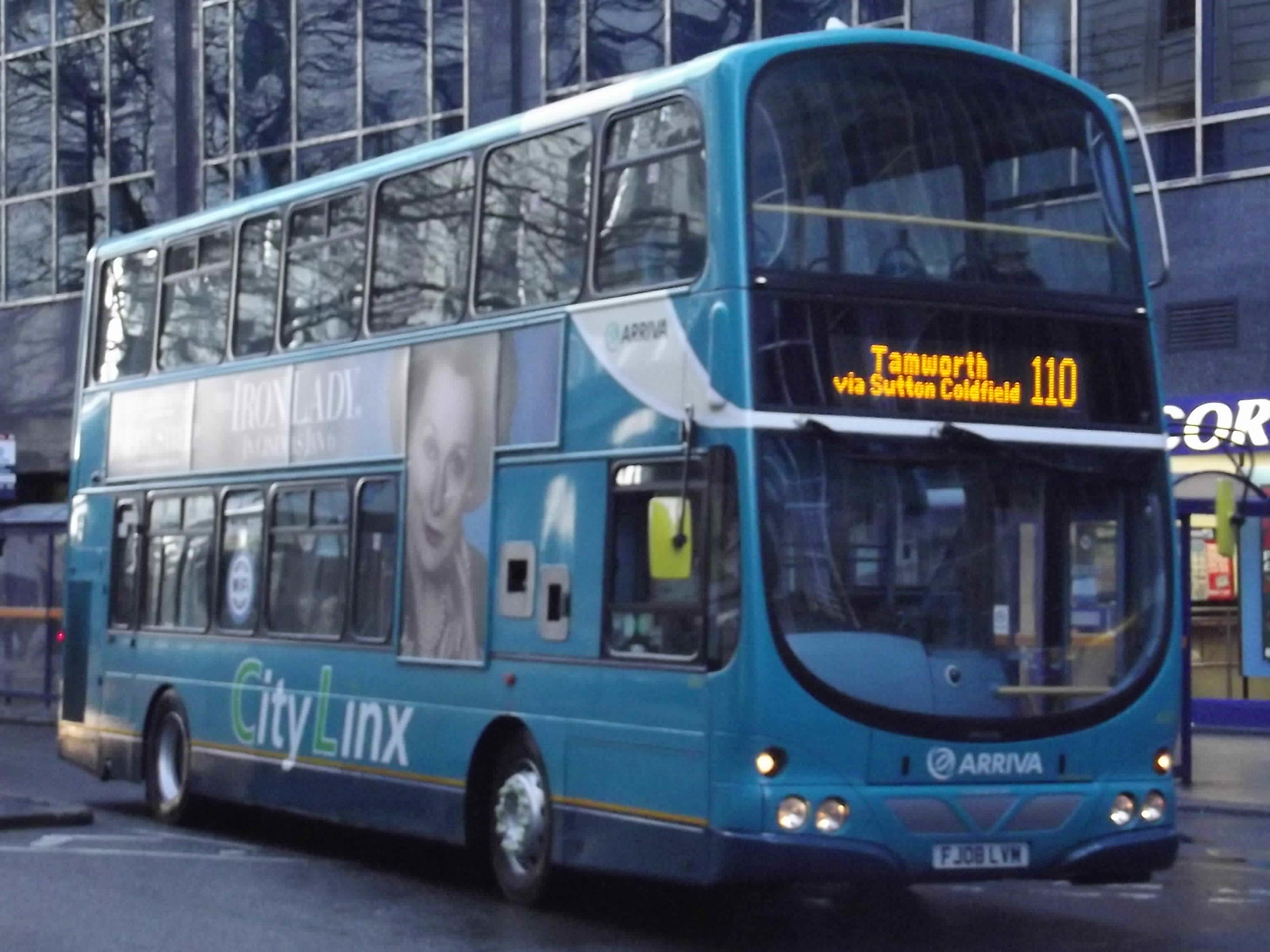This detailed photograph captures a blue double-decker bus named City Links, parked on a city street next to an office building with a similarly blue hue. Taken during twilight, the headlights of the bus are dimly illuminated, suggesting it might be sunrise or sunset. The bus features prominent front windows on both the lower and upper decks; through these, no passengers or drivers are visible.

On the side of the bus is an advertisement for the movie "The Iron Lady," featuring a black and white image related to the film. The bus's route information is displayed on a lit-up sign at the front, reading "Tamworth via Sutton Coldfield 110" in yellow lettering, indicating its destination and route number. The name 'Arriva' is inscribed below the front window, and the license plate reads FJOBLVM. The bus has gold trim near the tires, augmenting its sleek blue exterior.

In the background, there is a tall building with large windows and nearby shops, enhancing the urban atmosphere of the scene. The lack of bright lighting and the presence of multiple dimmed headlights reinforce the time of day, suggesting a bus ready to commence its journey through the city.